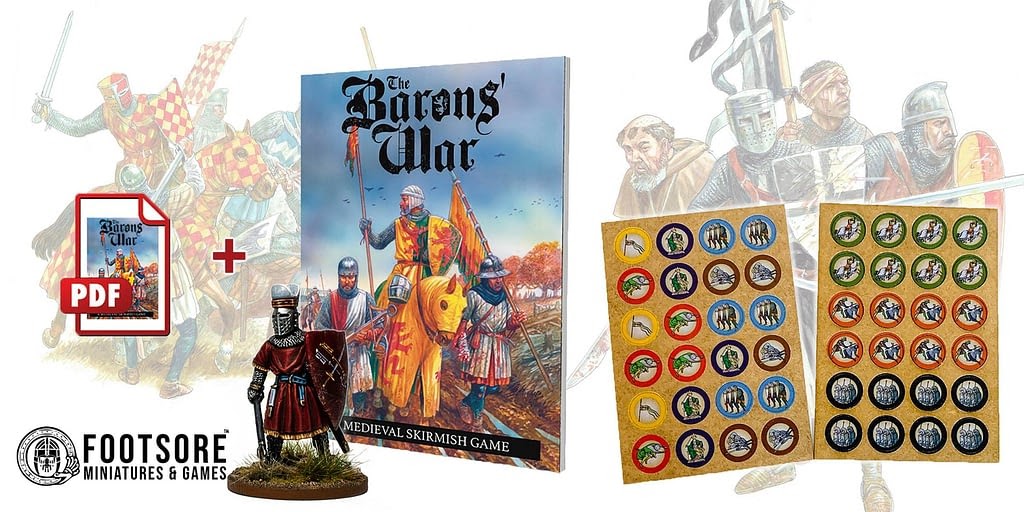This color photograph serves as an advertisement for a tabletop medieval skirmish game called "The Baron's War," produced by Footsore Miniatures and Games. The left portion prominently features the company's logo. In the foreground, a detailed miniature figurine of a knight is displayed, wearing a long red tunic, metal gloves, and holding a shield in his left arm and a sword in his right. The base of the figurine is textured with grass. 

Next to the miniature, a book is standing upright with "The Baron's War" emblazoned on the cover, along with depictions of two men marching beside a mounted knight. The book bears the subtitle "Medieval Skirmish Game." To the right of the book and the figurine, there are two sheets of colorful tokens or stickers, each adorned with various illustrations that relate to the game. In the background, a faded image depicts an intense medieval battle scene, with knights clad in vividly colored masks and armor, engaged in combat with swords and shields.

Additionally, the advertisement mentions that the game package includes both a PDF and a physical book, enriching the gameplay experience with comprehensive rules and additional content. The combination of these elements—the miniature, the book, the tokens, and the evocative medieval imagery—creates an immersive and visually striking representation of the game.